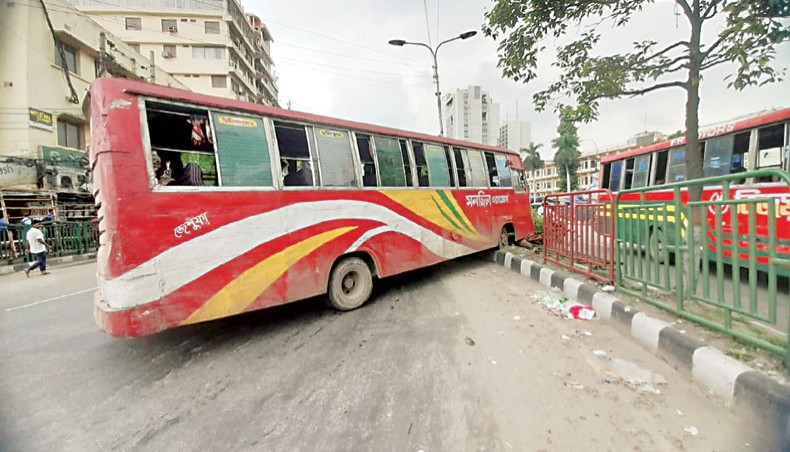The photograph depicts a city bus crash on a busy street, likely in India, judging by the writing on the bus which appears to be in an Eastern Indian script. The prominent red-and-yellow bus has veered off course, crashing through a center median, causing noticeable destruction. The median is lined with alternating red and green metal fencing, much of which has been knocked down due to the collision, revealing a striped gray and white concrete barrier beneath. In the midst of the wreckage, a street light, designed to light both sides of the road, stands tilted behind the bus. To the right of the fallen fencing, a similar bus matching the color scheme and design – including some white, yellow, and green leaf motifs – is either parked or driving by unscathed. The wheels of the crashed bus are noticeably dirty, and its open windows emphasize the sudden halt of its journey. The backdrop features residential and commercial buildings, including apartments and a hotel, while a damaged tree adds to the scene's chaos. Additionally, a pedestrian is seen on the left side of the road, examining the aftermath.